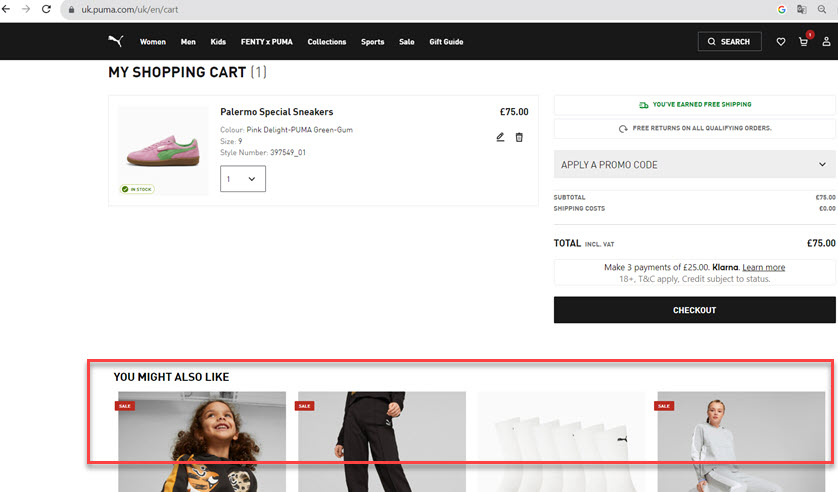This screen grab from the Puma UK website depicts a detailed view of the shopping cart page. At the top of the screen, the browser's gray address bar is visible, displaying the URL: "UK.puma.com/UK/EN/cart." Accompanied by a gray padlock icon, a refresh arrow, and a back arrow, the address bar also features a Google icon and a magnifying glass symbol.

Below the address bar, a black navigation bar is present with white text links to various categories: Women, Men, Kids, Fenty + Puma, Collections, Sports, Sale, and Gift Guide. Adjacent to this, there is a search box with a magnifying glass icon, a white heart icon, a shopping cart icon with a red notification circle, and a cartoon-like icon representing a user’s profile.

The main section of the page has a white background with the heading "My Shopping Cart (1)" written in black. Featured prominently is an image of a sneaker labeled "Palermo Special Sneakers" in the colors "Pink Delight" and "Puma Green," available in size 9. The shoe is priced at £75, and there are icons for editing (a pencil) and deleting (a trash can). A green box below the shoe image indicates that the item is "In Stock."

On the right side of the page, details about the order are outlined: "You've earned free shipping, free returns on all qualifying orders, apply a promo code." The subtotal is listed as £75, with shipping costs at zero, making the total, including VAT, £75. There is an option to "Make three payments of £25" through Klarna, with a link for more information, noting that it applies to those 18 and older and is subject to credit status. At the bottom of this section, there is a prominent black "Checkout" button.

Further down, the page displays images related to the sale items: a light-brown-skinned child with curly brown hair, a person's legs clad in black pants, a pair of white socks, and a model dressed in white. Each of these images is bordered by a red box, further drawing attention to these sale items.